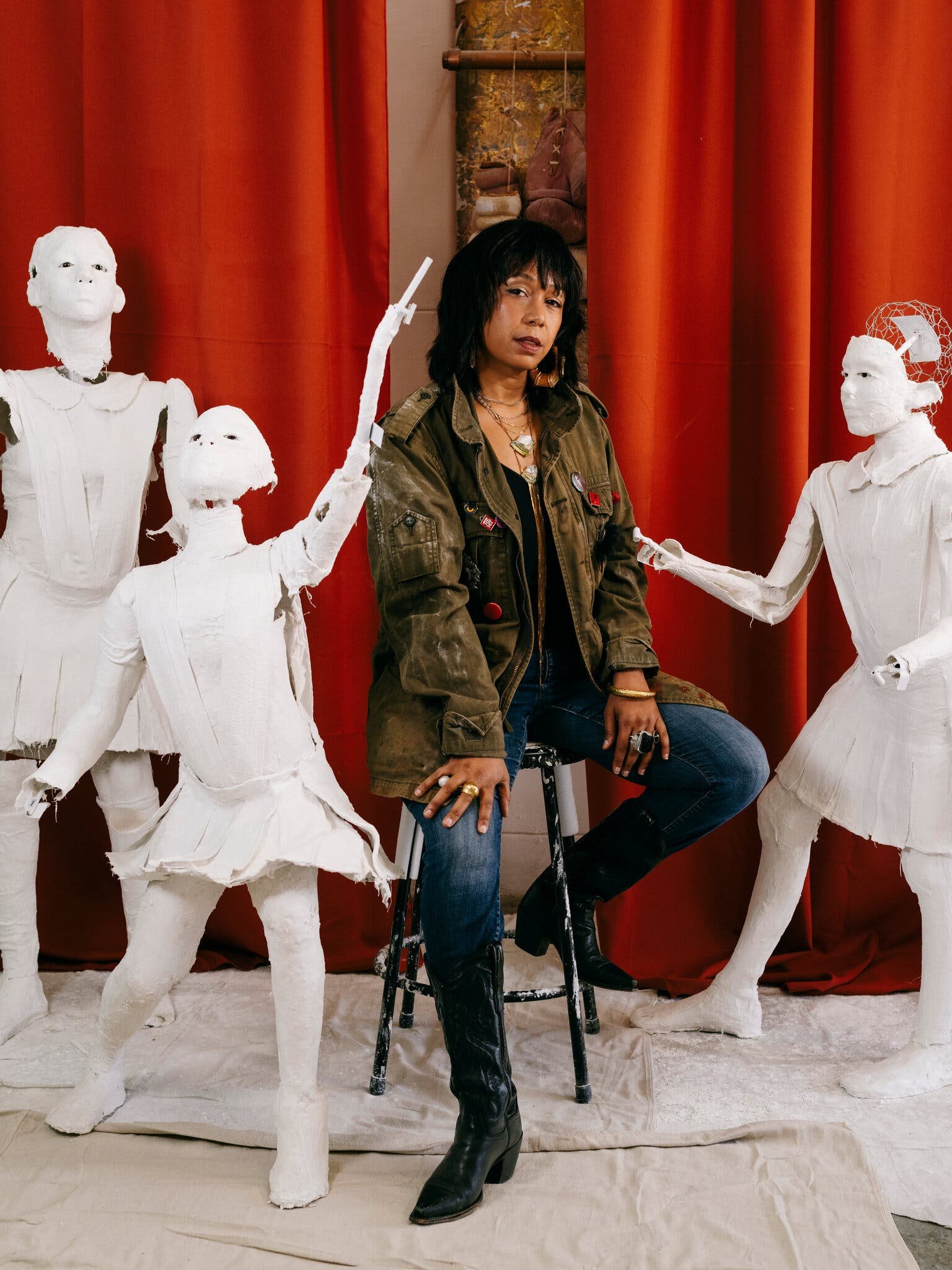In the photograph, a woman with dark tan skin and long black hair is seated confidently on a black stool, one foot resting on the stool's bottom rung and the other on the floor. She is dressed in an olive drab military-style jacket adorned with various colored pins and buttons, blue jeans, and black cowboy boots. Her jewelry consists of large gold hoop earrings, multiple necklaces, silver and gold rings, and a gold bracelet. Her demeanor exudes a daring, challenging presence as she faces the camera.

Surrounding her are three white mannequins made to look like plaster or papier-mâché, all missing their hands, replaced instead by stick-like protrusions from their wrists. The mannequins appear to be in dramatic movement poses; one resembles a little girl with a flared skirt and is posed with her arm raised, while another taller, more mature figure stands nearby. To the right, another mannequin seems to point towards the woman's head, her lifelike face and ear prominently visible.

The backdrop of the scene is a set of rich orangey-red curtains, partially open as if on a stage, with a white tarp or canvas covering the floor beneath, giving a theatrical and somewhat surreal atmosphere to the portrayal.